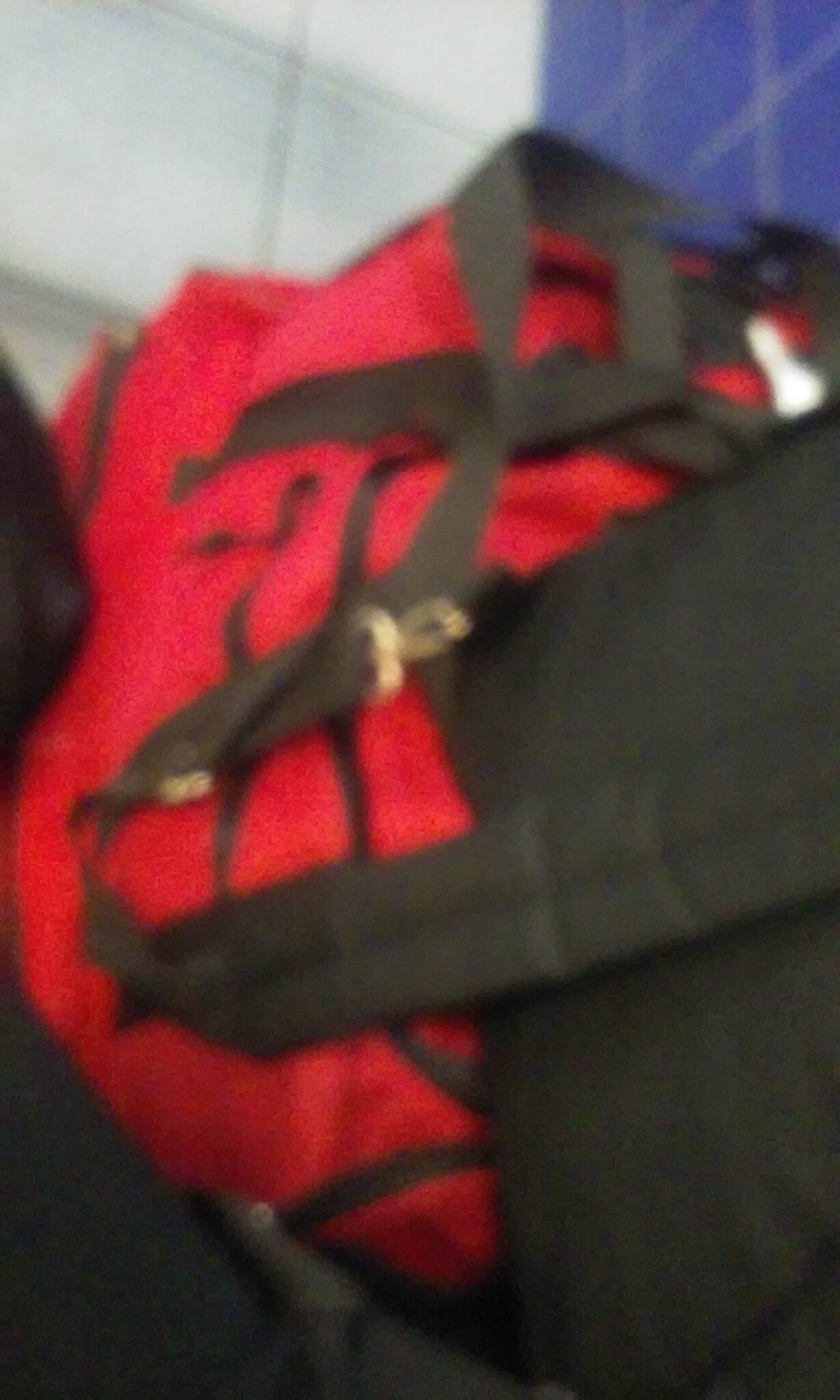The image is an exceedingly blurry and grainy photograph, seemingly taken by accident from a handheld phone, and depicted in a vertical orientation. It captures the corner of a room where two tiled walls meet: the left wall is adorned with large white tiles, while the right wall features smaller, bold blue tiles. In the center of the image lies a large black backpack, over which a red duffel bag, or possibly a life jacket, is draped. The red bag is detailed with black canvas straps, black zippers, and a bottom compartment with a zipper. A padded strap on the black backpack is visible, along with a gold clasp attached to a D-ring, indicating the presence of a crossbody bag. Additionally, another black object, resembling a backpack, extends into the image from the far-left side. The setup hints at a casual storage spot, possibly a shelf, where personal items like backpacks and jackets are temporarily placed.